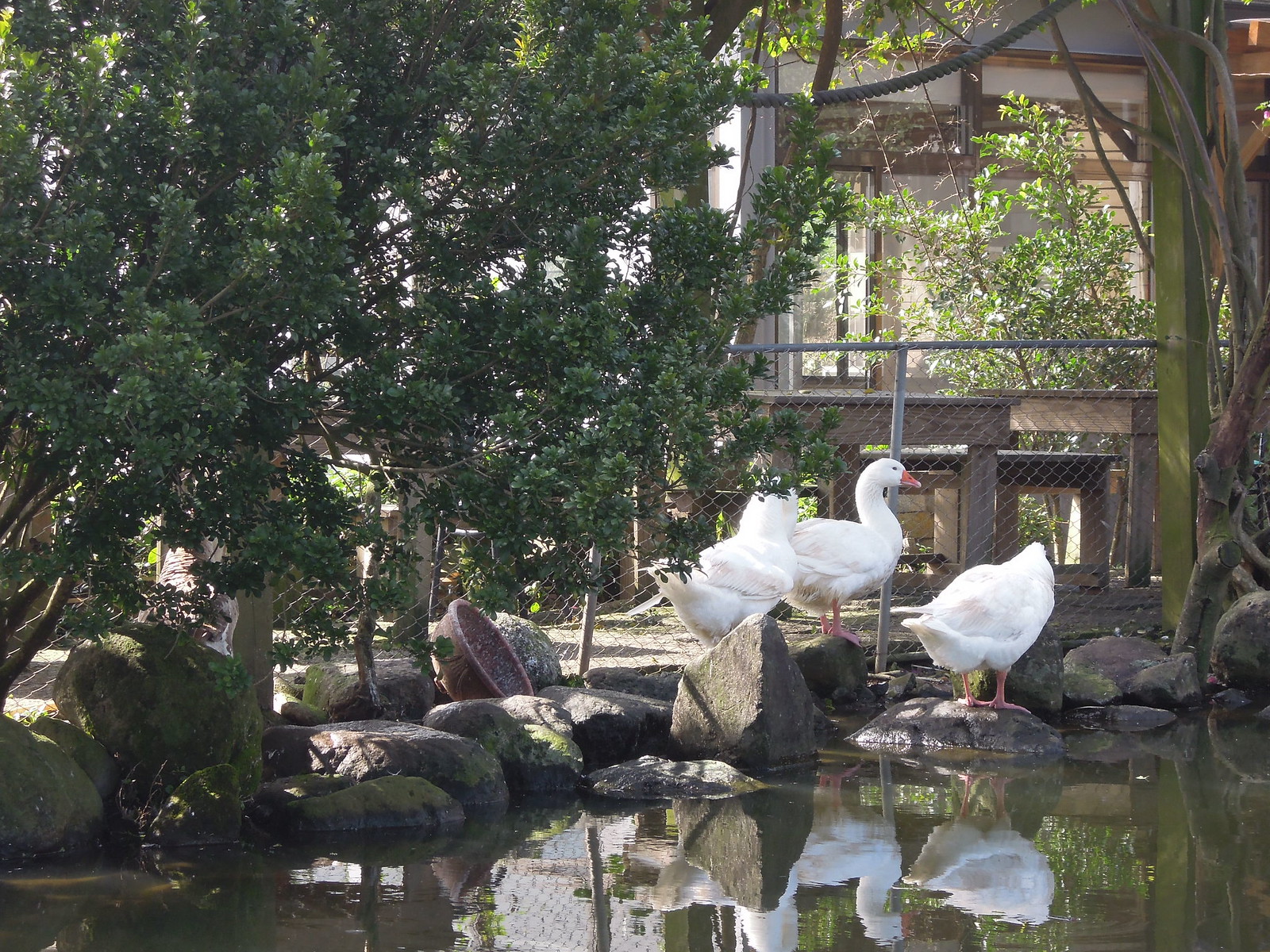The image captures three white ducks standing on gray, moss-covered rocks by the edge of a still pond. One duck is clearly visible in profile with an orange-red beak, while the other two have their bottoms facing the camera, obscuring their heads. The ducks are positioned slightly to the lower right of the center of the photograph. In the background, there's a chain-link fence enclosing the water feature, beyond which tables, benches, and indistinguishable wooden structures are visible. On the left side of the image, a large tree with lush green foliage is partially shown, with a scattered clay pot laying sideways on the rock. Various bowls and ropes are scattered around the pond area, adding to the scene's details. The overall setting is shaded and serene, with elements of greenery and man-made structures blending together.